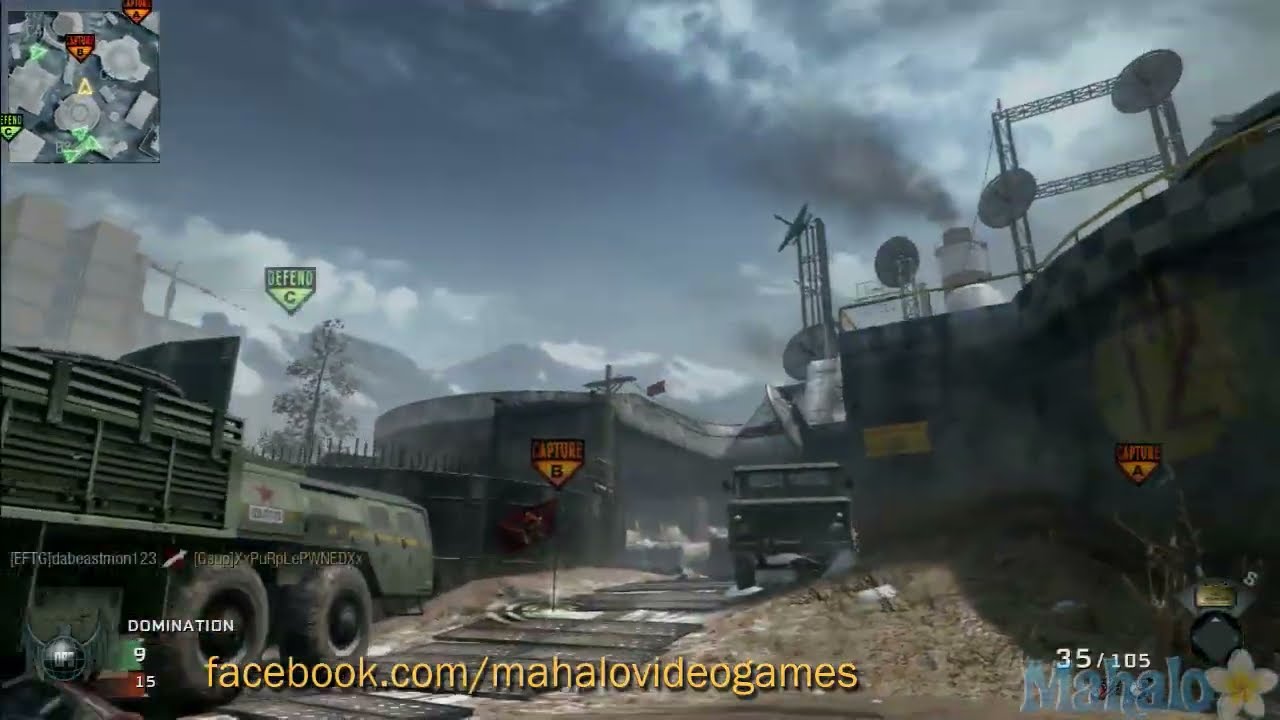The image is a detailed screenshot from a first-person shooter video game, reminiscent of Call of Duty, displaying an industrial, post-apocalyptic landscape. In the foreground, the player's left hand grips a large rifle, which features a distinctive red and black color scheme and a sight on top. The on-screen HUD indicates 35 out of 105 bullets remaining. The bottom of the screen prominently displays "facebook.com/MahaloVideoGames" in gold text, and another overlay in the lower right corner reads "Mahalo" with a small flower icon.

The central gameplay mechanics are visible, with "Domination" displayed in the lower left, showing a score of 9 (green) and 15 (red). Instructions to "capture B" and "defend" highlight objectives around the environment. The map in the upper left shows the player's position and objectives.

The setting is bleak and barren, with brown, desolate earth and a steely grayish-blue sky, absent of vegetation. A large vehicle resembling a tank and various industrial structures, including a large black fence with rebar, metal buildings with exposed weaponry, and a wall with spikes, populate the scene. The terrain features grates, a hill, and footprints amidst brown and black weeds. In the background, a concrete building and an elevated cab-like tractor underscore the dystopian atmosphere. Additionally, a greenish vehicle and a metal door are apparent near the structures, enhancing the detailed environment depicted in the game.